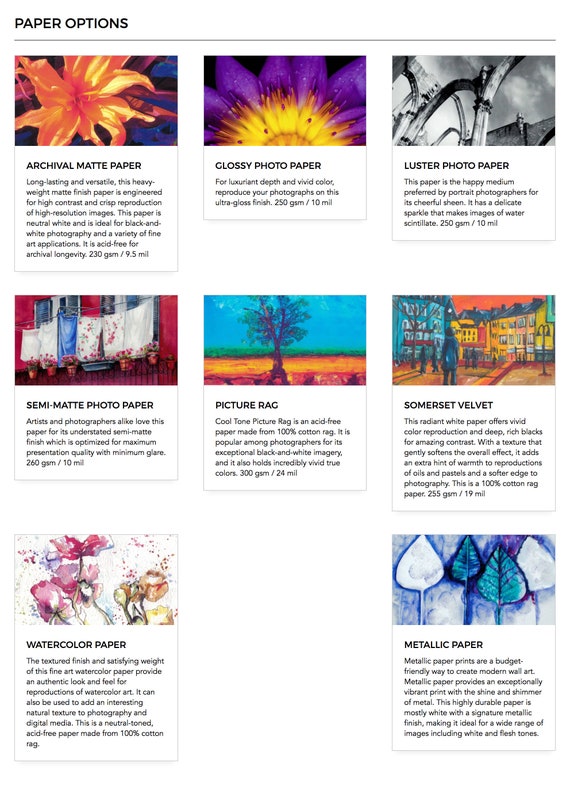This image, potentially a poster or advertisement, showcases a variety of paper options, titled "Paper Options" at the top. In three organized rows, each paper type is demonstrated through associated photographs or illustrations.

In the first row from left to right:
1. **Archival Matte Paper**: Features a vibrant color photograph of an orange daylily.
2. **Glossy Photo Paper**: Displays a colorful photograph of a purple passionflower.
3. **Luster Photo Paper**: Presents a black and white image of an unspecified subject.

In the second row:
4. **Semi-Matte Photo Paper**: Shows a vivid photograph, or possibly painting, of colorful laundry hanging outside balcony windows.
5. **Picture Rag Paper**: Highlights what appears to be a soft, impressionistic landscape painting, with touches of blue, orange, and green.
6. **Somerset Velvet**: Exhibits an acrylic painting of a bustling city street, rich in blues, yellows, and oranges, reminiscent of a European village scene.

In the third and final row:
7. **Watercolor Paper**: Features a delicate floral watercolor illustration with a white background.
8. **Metallic Paper**: Presents an abstract illustration of trees or leaves in a palette of blue, green, and silvery white.

Each paper type is depicted with a corresponding image to illustrate how prints would appear on the various paper options available. Small descriptive labels are situated beneath each image, completing the detailed showcase.